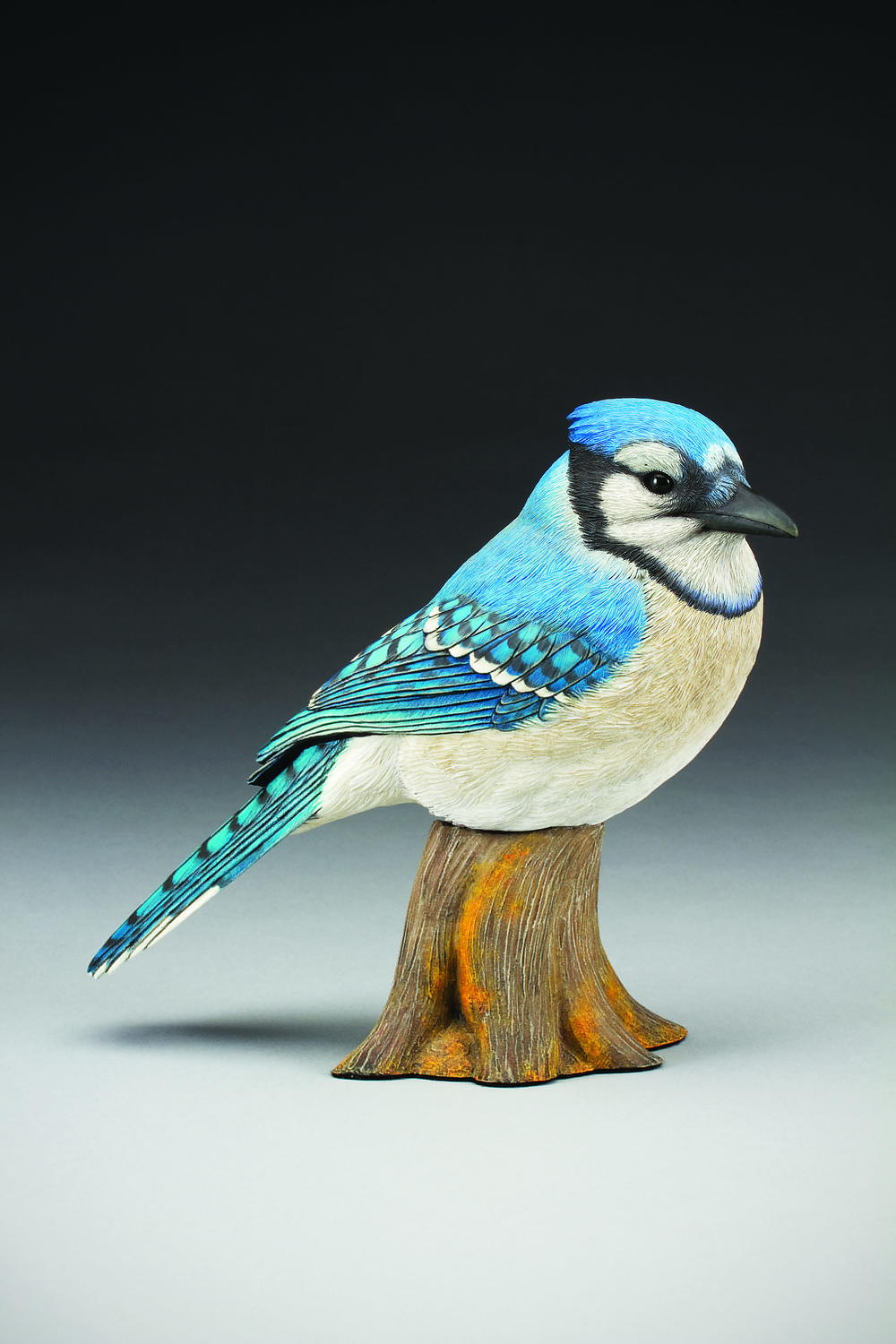This is an intricately detailed photo of a Blue Jay perched atop a small, sculpted tree stump. The bird, which appears to be a garden statue or possibly a stuffed Blue Jay, showcases the typical vivid blue feathers on its outer body, a blue tail, and a blue band over its head. Its beak and eyes are black, while its chest and belly are white with a touch of tan near the neck. Notably, there are black stripes over the eyes and delicate black lines interspersed within the blue feathers. The bird's positioning is such that it is facing towards the right-hand side of the image, and its wings are not spread, adding to the stillness of the scene. The backdrop of the photo is distinctive, featuring a gradient that transitions from dark black at the top to white at the bottom, creating a contrasting setting that highlights the bird and its shadow next to the tree stump.